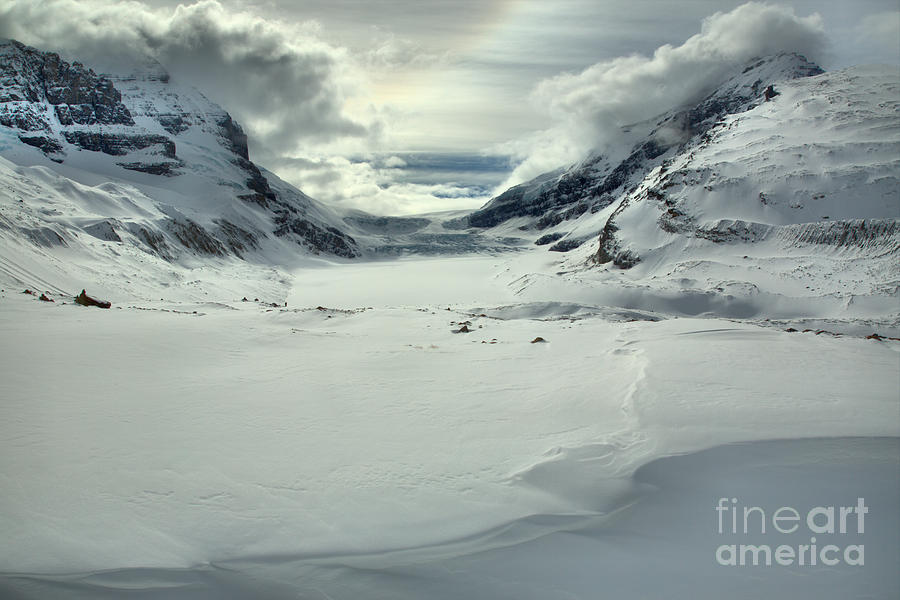This daytime photo captures a stark, wintry landscape dominated by two large, snow-covered mountains on the left and right. Nestled between them is a shallow valley, also blanketed in snow, which creates an almost entirely white and empty environment. The sky overhead is heavily clouded and gray, with fog or low-hanging clouds hovering above the mountain peaks. In addition to the pervasive snowy whiteness, small bits of rock and dirt can be seen peeking through the snow-covered ground, suggesting a rugged terrain. A body of water is visible in the background, adding depth to the scene. Unique to this otherwise monochromatic setting is a rainbow arcing gracefully across the cloudy sky, touching down near the mountain on the left. No signs of human presence can be found in this pristine, natural landscape. At the bottom right corner of the image, the text "Fine Art America" is subtly inscribed in light gray, marking the photo's artistic attribution.